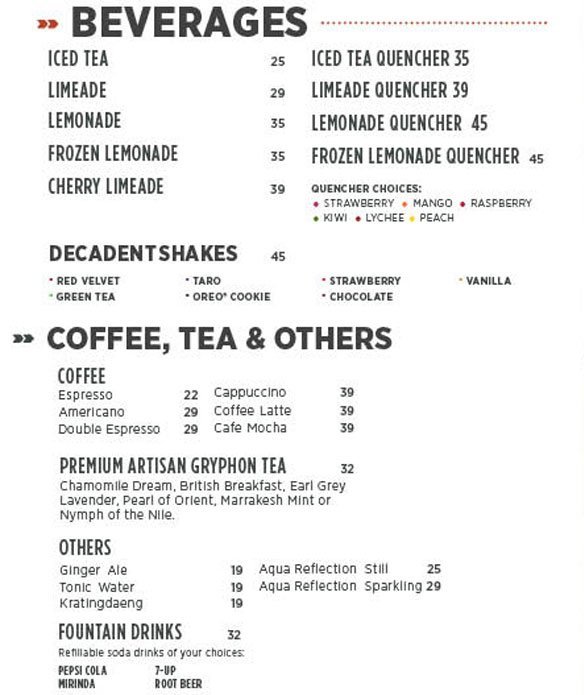The image depicts a detailed beverage menu with various drink options, presented on a white background with black lettering. The menu lists an extensive selection ranging from basic beverages like iced tea ($25), limeade ($29), and fountain drinks such as Pepsi, Cola, and 7-Up ($32), to more intricate offerings. Unique items include frozen lemonade quenchers, decadent shakes with flavors like Red Velvet, Oreo Cookie, and Taro, and a range of coffee options such as espresso ($22), cappuccino ($39), and café latte. Additionally, the menu features premium artisanal Griffin tea, tonic waters, ginger ale, and sparkling aqua reflection. The prices suggest that the currency is not U.S. dollars, indicating that this is likely a foreign menu.